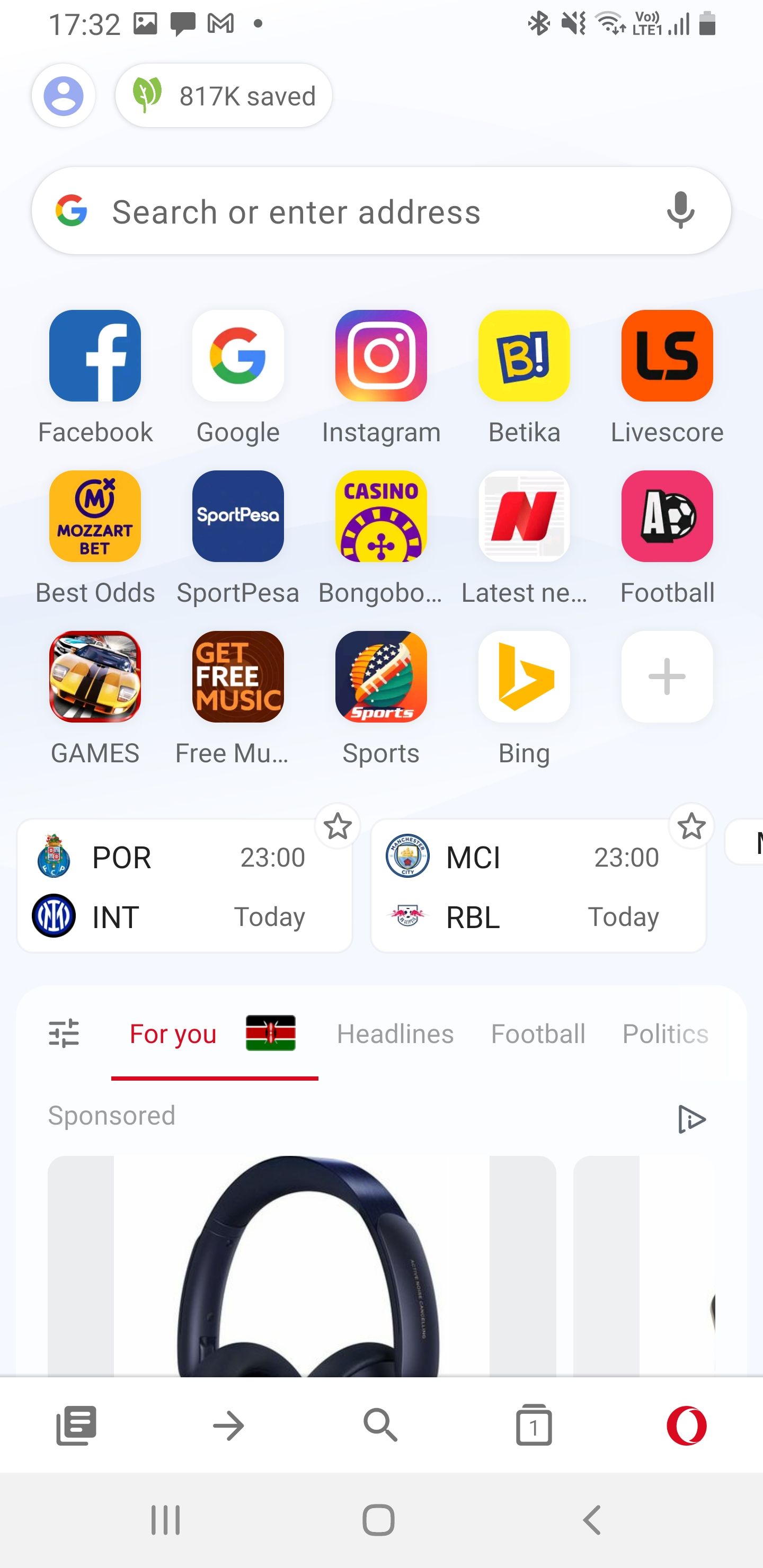The top center of the image features a search box that reads "Search or enter address," specifically designed for Google searches. Below the search box, an array of app icons is displayed in a neatly organized grid:

- **Facebook:** Blue and white icon.
- **Google:** White icon with a multi-colored "G" in red, yellow, green, and blue.
- **Instagram:** Icon with a gradient of purple, orange, and white.
- **Betica:** Yellow icon with a "B" outlined in blue.
- **LiveSchool:** Orange icon with "LS" written on it.
- **BestOdd:** Yellow icon with "MozartBet" written on it.
- **SpotPesa:** Blue icon with "SpotPesa" written in white.
- **BongoBongo:** Yellow icon with "Casino" written on it.
- **LatestNews:** White icon with a red edge.
- **Football:** Pink icon with an "A".
- **SoccerBall:** Icon not described, presumably related to soccer.
- **Games:** Icon featuring a car image.
- **FreeMusic:** Icon with "Get Free Music" text.
- **Spots:** Icon showing a design with spots.
- **Bing:** Yellow icon with the Bing logo, which is a stylized "B".

At the bottom of the image, there are two sections highlighting sports matches:
- On the left side: A match between Portugal and Inter Milan scheduled for 23:00 today.
- On the right side: Another match between Manchester City and Real Betis also scheduled for 23:00 today.

Below these sections, there are categorized sections labeled "For You," "Headlines," "Football," and "Politics." At the very bottom, there is a piece of sponsored content advertising black headsets.